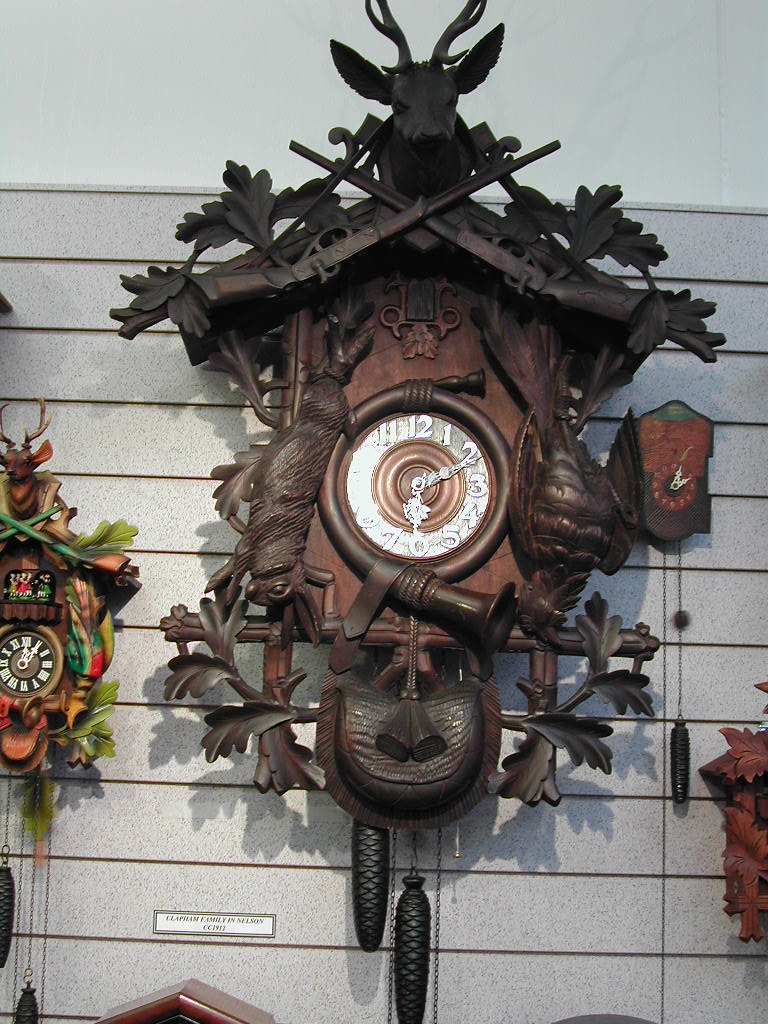The image showcases a collection of intricately designed cuckoo clocks. The focal point is a particularly large and ornate clock situated in the center. This prominent timepiece features a clock face in the center, adorned with white numerals and hands, contrasted by a golden center. Encircling the clock face is a beautifully crafted miniature house, embellished with an abundance of detailed leaves and intertwining vines, creating a rich tapestry of nature-inspired elements.

Dangling from the bottom of the clock are the traditional cone-shaped weights, essential for regulating the clock's timekeeping mechanism, attached by delicate cords. 

To the left of the central clock, there is a medium-sized cuckoo clock, slightly less elaborate but still remarkable in its craftsmanship. On the right side, a very tiny cuckoo clock adds charm to the collection, providing a striking size contrast within the display. The array of clocks collectively highlights the artistry and meticulous attention to detail inherent in these timeless pieces.